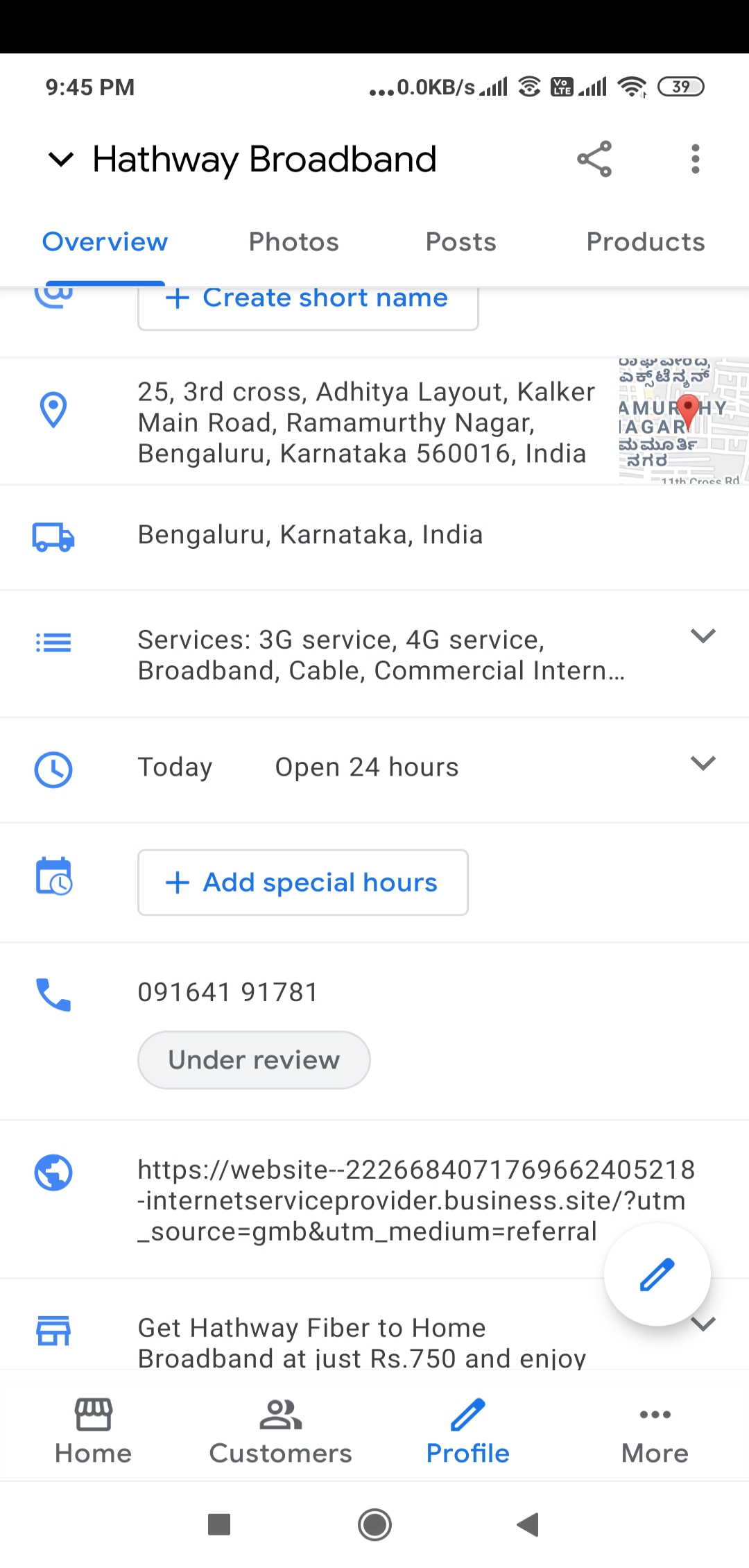Here is a cleaned-up and detailed caption for the given image:

---

The image depicts a smartphone screen showcasing the user interface of an app or webpage. At the top, there is a black status bar displaying the time, "9:45 p.m.," followed by a sequence of indicators. From left to right, the indicators show an ellipsis (…), "0.0 KB/s," four 5G signal bars, a Wi-Fi signal icon, a telephone icon, and another set of four signal bars indicating LTE connection. This segment concludes with a battery status icon displaying "39%."

Below this status bar, the interface is divided into various sections starting with a navigation panel featuring an arrow pointing downwards labeled "Hathaway Broadband." To the right, there is a share icon and another ellipsis. The horizontal navigation menu lists tabs such as "Overview," "Photos," "Posts," and "Products," with the "Overview" tab highlighted and underlined in blue.

The detailed content of the "Overview" section is organized as follows:
1. An initial entry slightly cut off that includes a logo and an option to create a short name.
2. A pin icon with the text "25."
3. Address details, including "Adhita Layout, Cow Curve Main Road, Rama Murti Nagar, Bengaluru, Karnataka, 560016, India," with a small map pin icon by its side.
4. A blue truck icon next to the location "Bengaluru, Karnataka, India."
5. A triple-line icon listing various services ("3G service, 4G service, Broadband cable commercial internet...") with a dropdown arrow.
6. A blue clock icon stating "Today" and "Open 24 hours" with another dropdown arrow.
7. A calendar icon detailing special hours with an option to add new special hours.
8. A blue telephone icon with the number "09164 19178," followed by an "Under review" button.
9. A globe icon and a long URL: "https://website-2266840717696240521-internet-service-provider.business.site/?utm_source=GMB&utm_medium=referral."
10. A house icon with the promotional message, "Get Hathaway Fiber to Home Broadband at just RS 0.750 and enjoy."

At the bottom, the screen has a small navigation bar featuring options such as "Home" with a business icon, "Customers" with a people icon, "Profile" with a pin icon (highlighted in blue), and "More" with an ellipsis.

Finally, beneath this navigation bar, there are additional icons for the phone's user interface, including a square, a circle, and an arrow pointing to the left.

---

This revised caption encompasses all the essential elements and details from the original description, making it more structured and easier to understand.